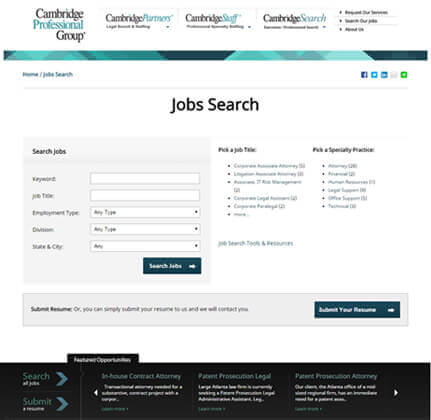A detailed caption for the given image would be:

"The image features a predominantly white background with the title 'Cambridge Professional Group' displayed at the top in bold letters. Beneath, there are three subheadings: 'Cambridge Purposes,' 'Cambridge Stuff,' and 'Cambridge Search,' each marked with an asterisk beside them. Central to the image is a blue and black rectangular box containing various elements related to job search functionalities. A smaller box within this section displays icons for Facebook and Twitter, suggesting integration with social media.

There is a horizontal line labeled 'Job Search' and below it, a prominent blue box that reads 'Search Jobs.' This box includes input fields for entering your name and job title. To its right, dropdown menus labeled 'Pick a Job Title' and 'Pick a Specialty' allow users to refine their job search criteria. 

At the bottom of the image, a blue stripe houses a 'Submit Resume' option, accompanied by a button to upload or submit your resume. The bottom-most section features a black box with blue arrows pointing to the right, possibly indicating further navigation options."